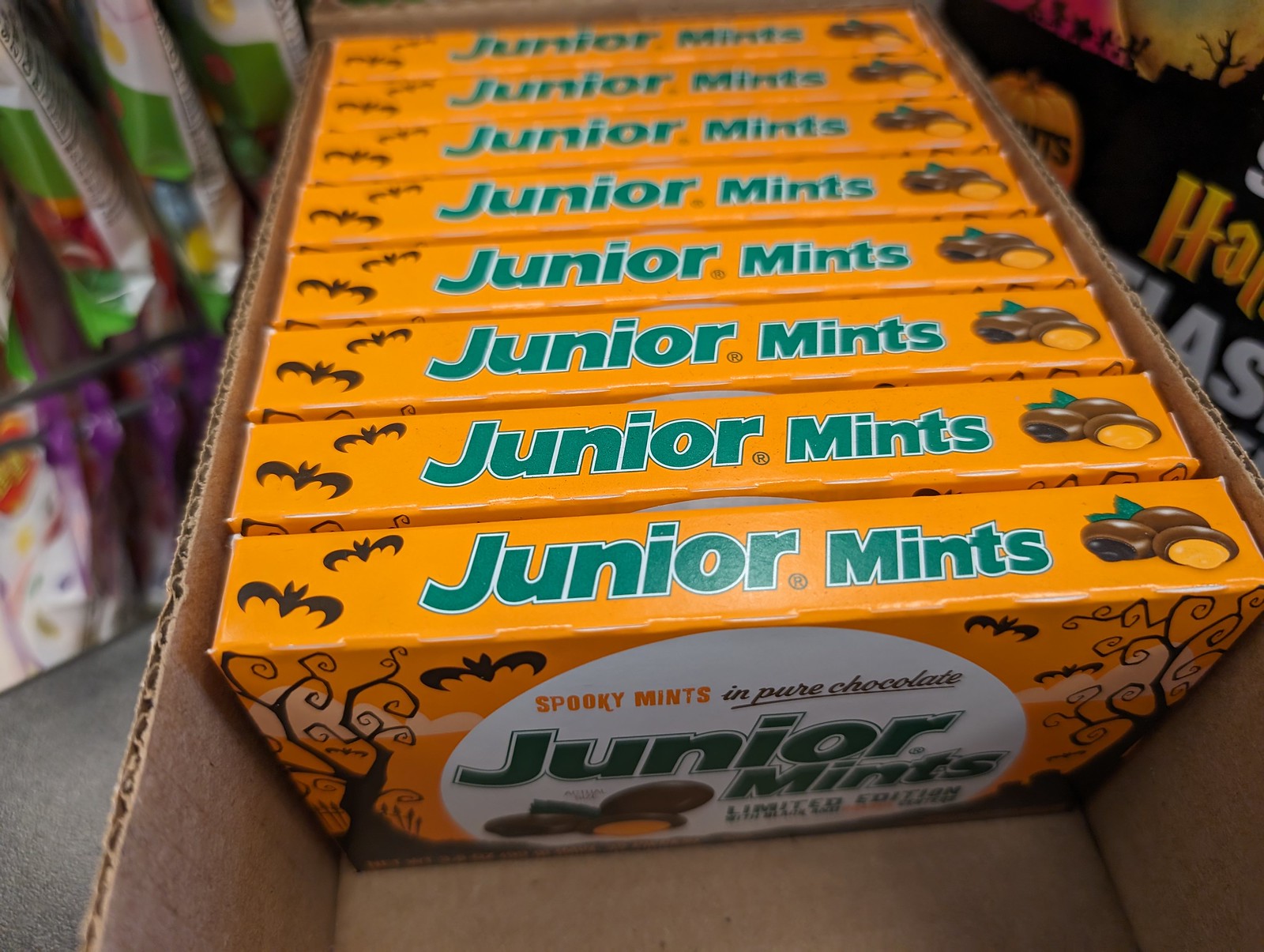This full-color image captures a brown cardboard box containing approximately eight rectangular boxes of Halloween-themed Junior Mints. Each smaller box is orange with detailed seasonal artwork, featuring black bats and spooky, twisty trees, set against a white background. The prominent text on the boxes reads "Spooky Mints in Pure Chocolate," with "Spooky Mints" in eye-catching orange and "in Pure Chocolate" in brown. An illustration of the mints shows them with red, orange, and black fillings instead of the typical white, emphasizing the Halloween theme. In the background, there is more Halloween decor, including a sign that says "Halloween" in orange on a black background and a pumpkin, suggesting this photo was taken in a store during the Halloween season.